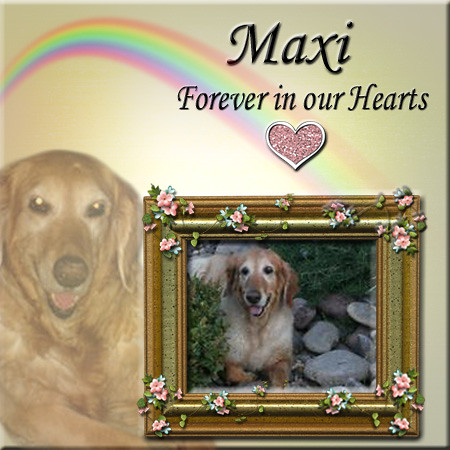This commemorative card for a deceased dog named Maxi features a square design with a yellowish background and a prominent rainbow arching from the top left to the bottom right. The card's title "Maxi" is displayed in large letters at the top, followed by the touching phrase "forever in our hearts" in elegant script. Below the text is a heart shape, adorned with a golden border and filled with pink, sparkly glitter.

In the lower right portion of the card, a framed photograph of Maxi as a golden retriever is showcased. The picture frame is gold with decorative pink and green flowers and leaves sprinkled around the edges, surrounding an image of Maxi lying on the grass beside some large cobblestone rocks. To the left of this framed picture, a slightly translucent, superimposed image of a younger Maxi is embedded into the card, adding to the sentimentality of the memory. The overall card design evokes a sense of heartfelt remembrance, showcasing the beloved dog's image against a backdrop rich with color and emotion.